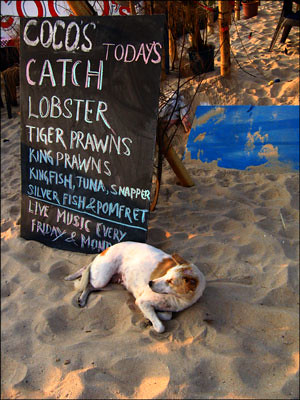In this detailed beach scene, a white dog with brown markings on its head lays comfortably in the sand, with its paws folded in front. Beside the dog, there is a prominent black chalkboard sign with white lettering that reads "Coco's Catch, Today's Catch: Lobster, Tiger Prawns, King Prawns, Kingfish, Tuna, Snapper, Silverfish," and advertises "Live Music Every Friday and Monday." The sign is upheld by a brown chair and is accompanied by various background elements, including a blue raft-like object positioned near another chair, a potted plant, a red and white sign, and the lower halves of several tiki statues. Electrical wires are visible in the backdrop, hinting at a potential setup for live music, aligning with the advertised entertainment.